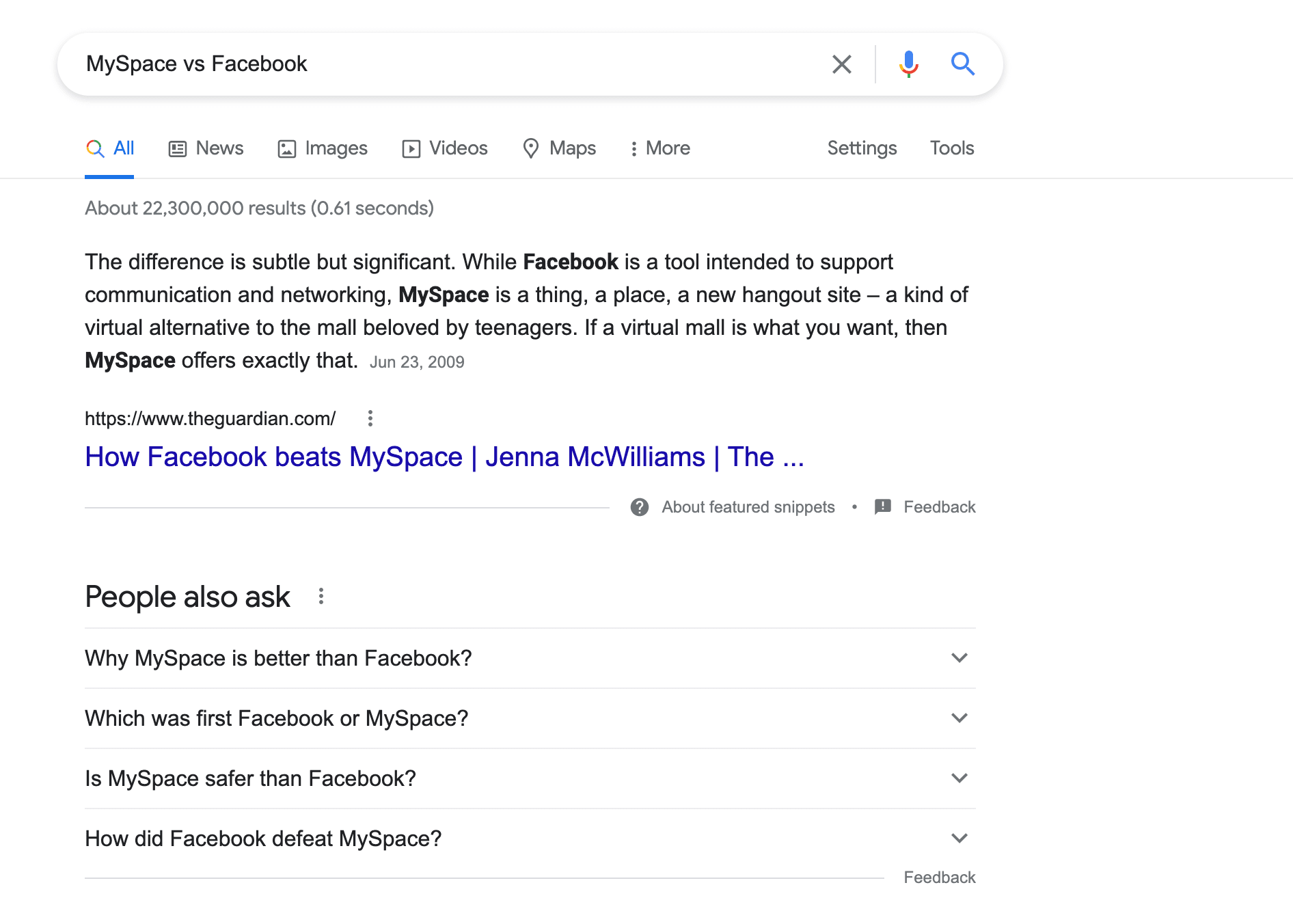The image captures a screenshot of a Google Chrome browser displaying search results for the query "MySpace versus Facebook." At the top, a search field is visible with the query typed in black font. Just below the search bar is a menu with options including "All," "News," "Images," "Videos," "Maps," "More," "Settings," and "Tools," with the "All" tab selected.

Further down, there is an indication of the total number of search results, shown as "About 22,300,000 results (0.61 seconds)" in gray font. The top search result is highlighted, featuring a detailed comparison of Facebook and MySpace. The result reads:

"The difference is subtle, but significant. While Facebook is a tool intended to support communication and networking, MySpace is a thing, a place, a new hangout site, a kind of virtual alternative to the mall beloved by teenagers. If a virtual mall is what you want, then MySpace offers exactly that."

This entry is dated June 23, 2009, attributed to Jenna McWilliams, and sourced from theguardian.com. Below this description, the section "About Featured Snippets" and a "Feedback" option are provided in gray font.

Further down in the screenshot, the "People Also Asked" section is visible, featuring related questions such as "Why is MySpace better than Facebook?", "Which was the first, Facebook or MySpace?", "Is MySpace safer than Facebook?", and "How did Facebook defeat MySpace?" Each of these questions is presented in black font, inviting users to explore more information.